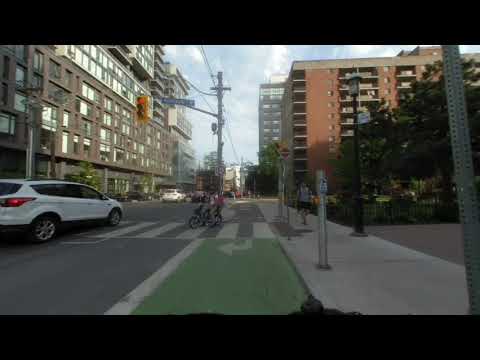In a bustling urban environment, this image captures a scene at a one-way street intersection marked by a red traffic light. A white SUV is stopped improperly in the crosswalk, causing two cyclists to wait behind it. The crosswalk intersects a bright lime green bike lane, distinct from the grey asphalt road. Surrounding the scene are towering city buildings: a very large brown building with numerous windows on the left, and two more brown buildings with balconies on the right, extending towards the horizon. Further down the sidewalk on the right, a parking meter is positioned within a green-painted zone marked with an arrow. The sky above is a light blue with few clouds, indicating a sunny day. A man is walking down the grey concrete sidewalk towards the camera, and scattered throughout the scene are poles, streetlights, and hints of trees and possibly a small park area, adding to the urban landscape.